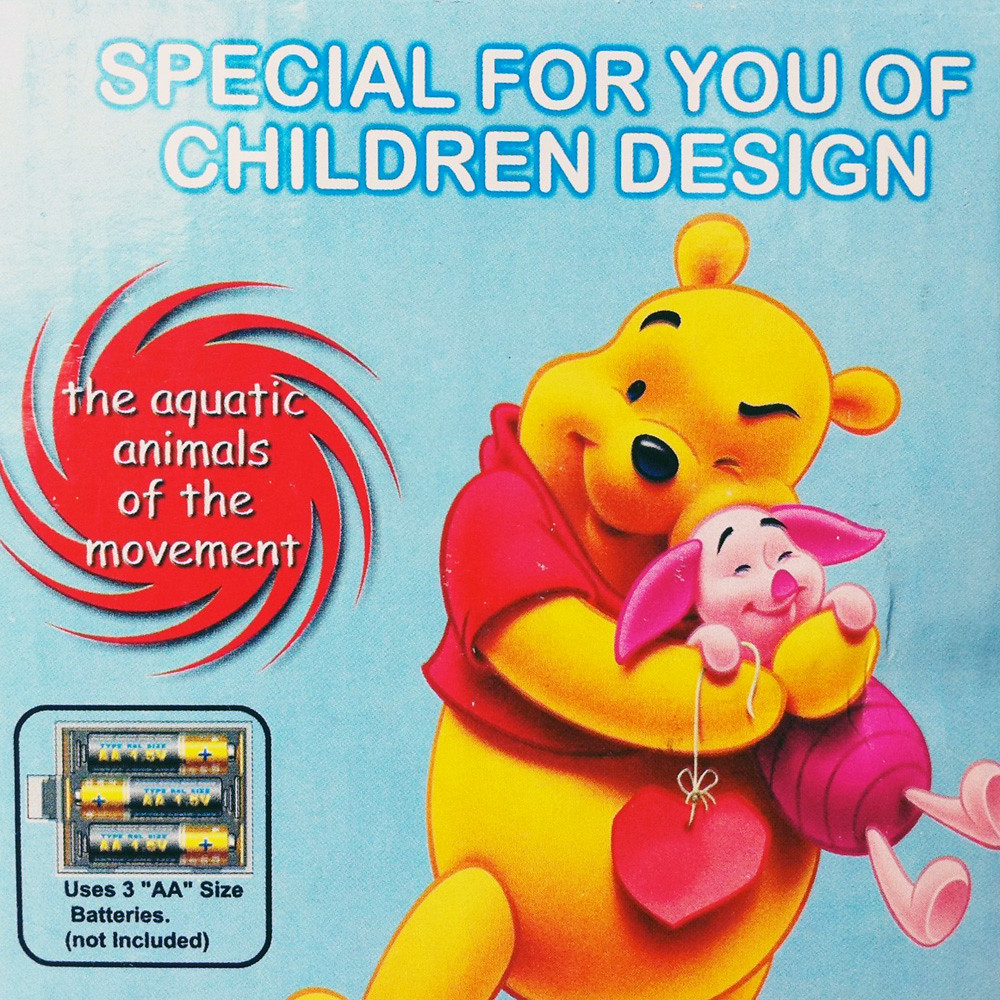This image features a light blue background with a prominent cartoon depiction of Winnie the Pooh and Piglet in the center. At the top of the image, bold white bubble letters outlined in blue read, "Special for You of Children Design." Positioned to the left of Pooh and Piglet is a red, swirly medallion resembling a whirlpool, containing the text in white, "The Aquatic Animals of the Movement." Below this medallion, there is a black square with rounded corners illustrating the placement of batteries, accompanied by the text, "Uses three AA size batteries, not included." Winnie the Pooh, depicted as a bright yellow bear with a red shirt, is hugging Piglet, who appears in varying shades of pink. Piglet holds a white string from which a big red paper heart dangles.